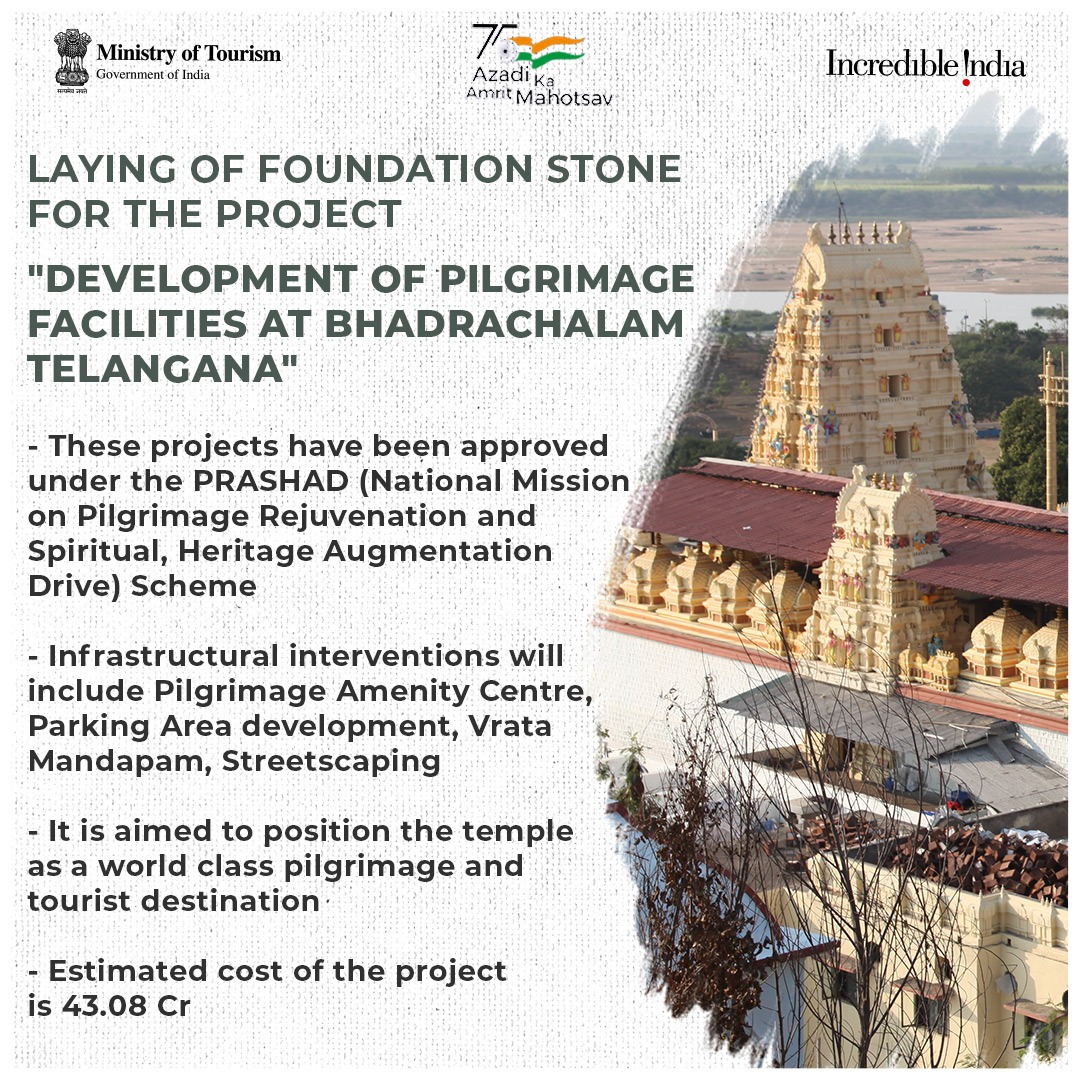This intricate promotional image from the Ministry of Tourism, Government of India, boasts a detailed and comprehensive advertisement designed to highlight the development of pilgrimage facilities at Badrachalam, Telangana. Set against a textured white background, the upper segment of the image features the Ministry's emblematic logo beside the official title, accompanied by text in Hindi, and the prominent tagline "Incredible India." The core of the advertisement outlines the recently approved projects under the PRASHAD (Pilgrimage Rejuvenation and Spiritual Heritage Augmentation Drive) National Mission, aimed at transforming the temple area into a world-class pilgrimage and tourist destination. The infrastructural enhancements mentioned include pilgrimage amenities, a century parking area, Vrata Manipan, and streetscaping, with an allocated budget of 43.0 ACR. Complementing the text is a vibrant image on the right depicting Indian architectural marvels, including tan pyramids, a building with a maroon roof and numerous tables, surrounded by lush greenery, further emphasizing the locale's cultural richness.